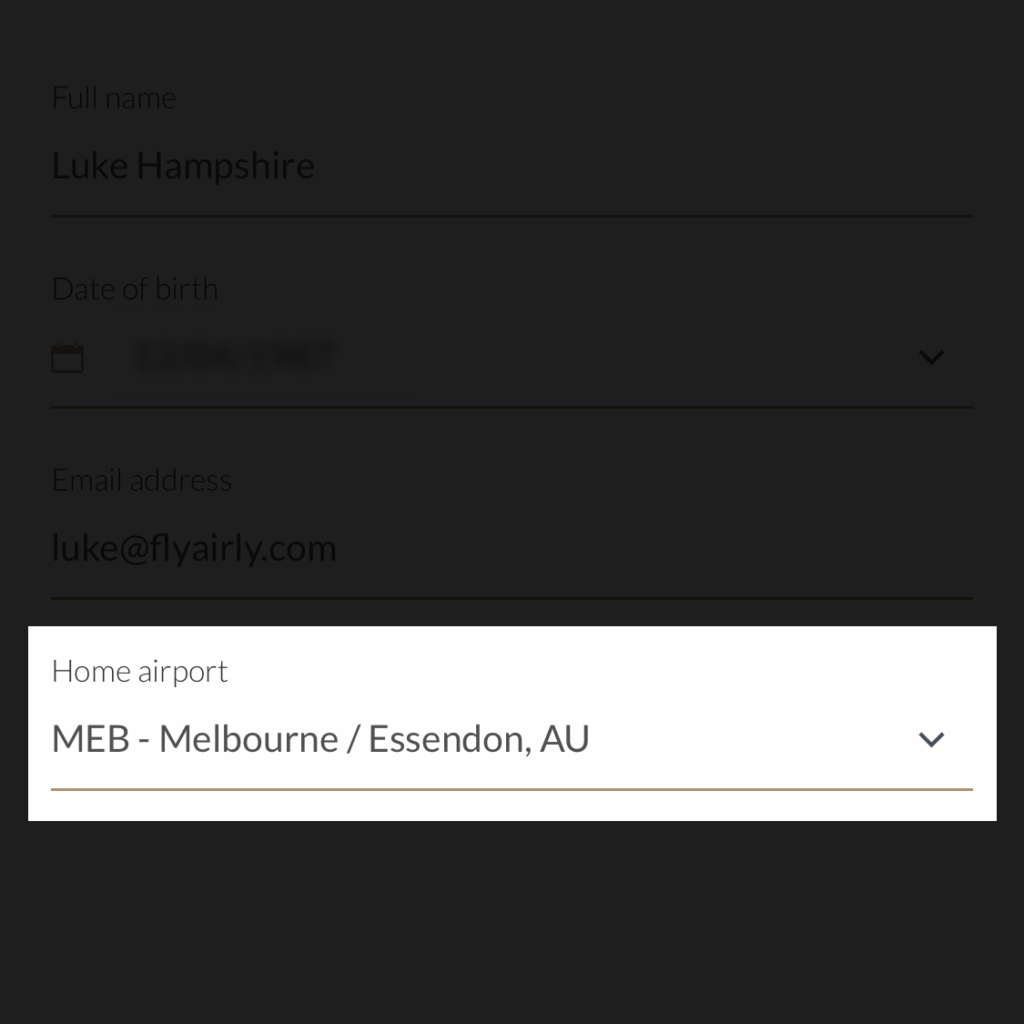The image showcases a digital screen, likely from a phone or computer, with a black background filled with faint words and rectangular sections. Prominently displayed is a popup window positioned about three-fourths down the screen. The background text includes fields such as "Name: Luke Hampshire," "Date of Birth," and "Email Address." The popup window features a gray header titled "Home Airport," followed by a drop-down menu. The selected option in the menu is "MEB - Melbourne/Essendon, AU," accompanied by a drop-down arrow to its right. Beneath this menu is a brownish line that adds a subtle division. The lower part of the screen appears obscured by a dark overlay, concealing some background elements.